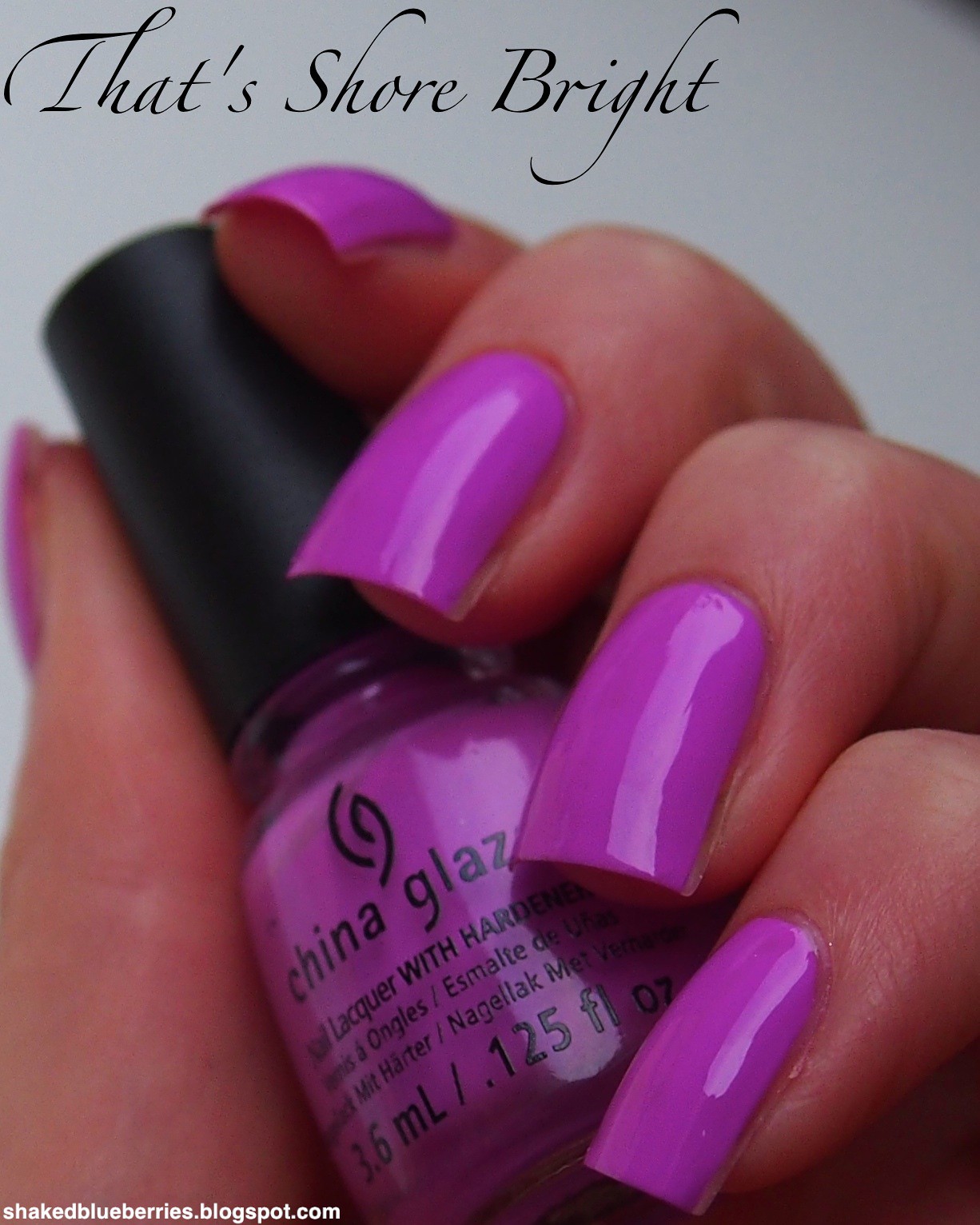The image is a detailed advertisement for a nail salon or nail polish company, featuring the brand China Glaze. Set against a slate gray background, it displays a close-up of a woman's left hand, which is the focal point. Her nails are painted in a vibrant lavender purple, identical to the color of the nail polish bottle she is holding. The hand is positioned with fingers slightly bent, gripping the bottle, which is tilted obliquely. The nail polish bottle is made of clear glass with a tall black lid, and features a leaf logo along with the brand name "China Glaze" in black lettering. Additional text on the bottle mentions that it is a "soft lacquer with hardener" and indicates the volume as 3.6 ml / 1.25 fl oz. At the very top of the image, in bold black lettering, is the phrase "That's Sure Bright." In the bottom-left corner, a white text overlay reads "shakedblueberries.blogspot.com."